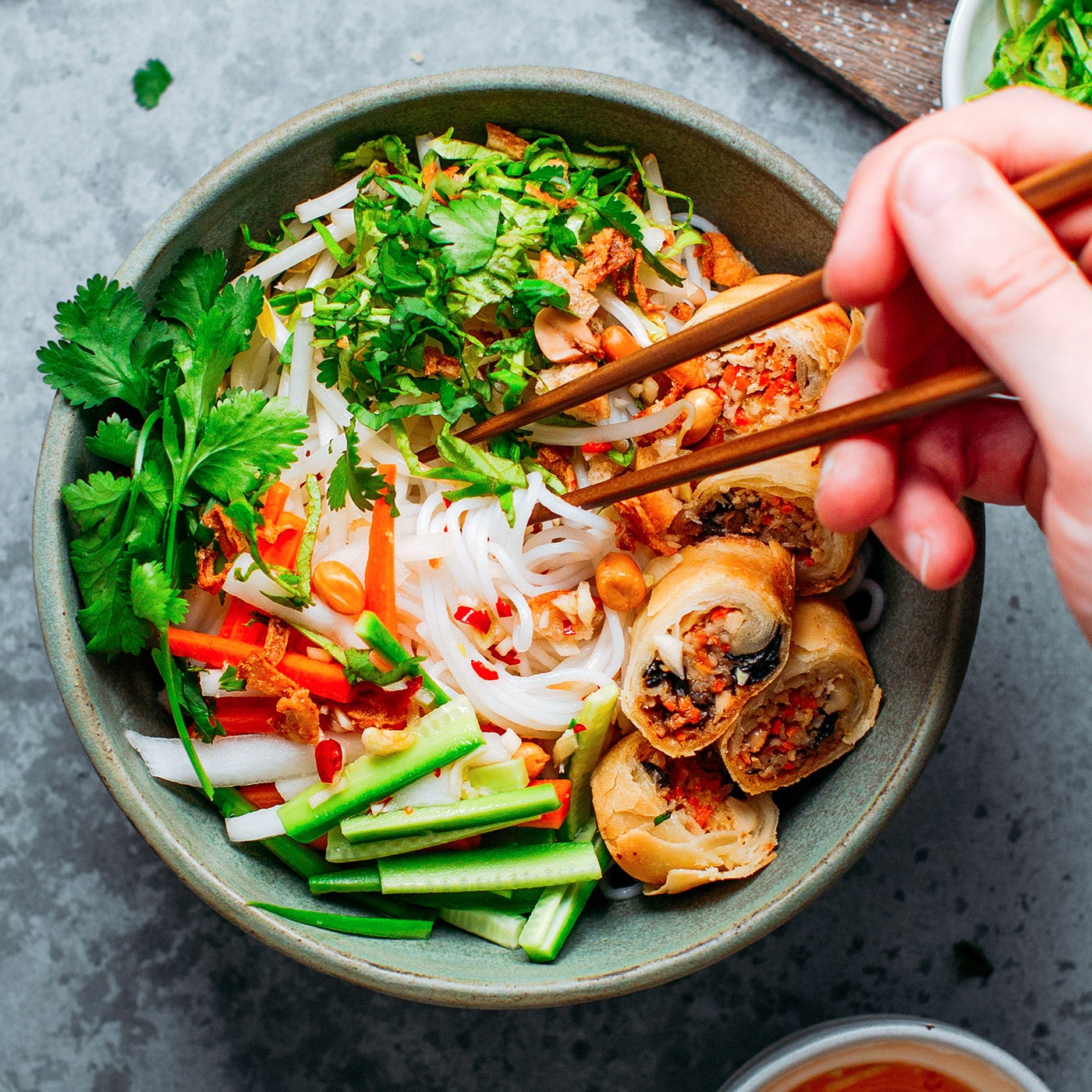The photograph showcases a delectable meal presented in a speckled gray ceramic bowl, positioned on a metallic gray, spotted table. Captured from a top-down angle, the image prominently features a slightly blurry hand in the upper right corner, likely a man's, gripping a pair of medium brown chopsticks with the thumb over the top and fingers wrapped below. The chopsticks are poised above a medley of enticing ingredients within the bowl.

At the center of the bowl, a nest of white rice noodles sits, surrounded by a variety of fresh and colorful foods. There are sliced zucchini or cucumber at the bottom and vibrant green parsley leaves on the left. Nestled among the noodles are small, fried items that could be egg rolls, evident from their golden-brown hue and an assortment of visible fillings that include red, black, yellow, and brown colors. The veggies include potentially cut celery, further complemented by scattered herbs and seeds. 

To the bowl's right side, additional noodles and a portion of some leafy greens extend towards the rim. In the lower right corner of the photograph, a small, white condiment container filled with red sauce sits, ready to enhance the dish's flavors. Further details include a cutting board in the upper right with a small bowl containing salt and more herbs, contributing to the overall gourmet aesthetic. The light source illuminating the scene emanates from the upper left, adding a pleasing highlight to the meticulously arranged food.